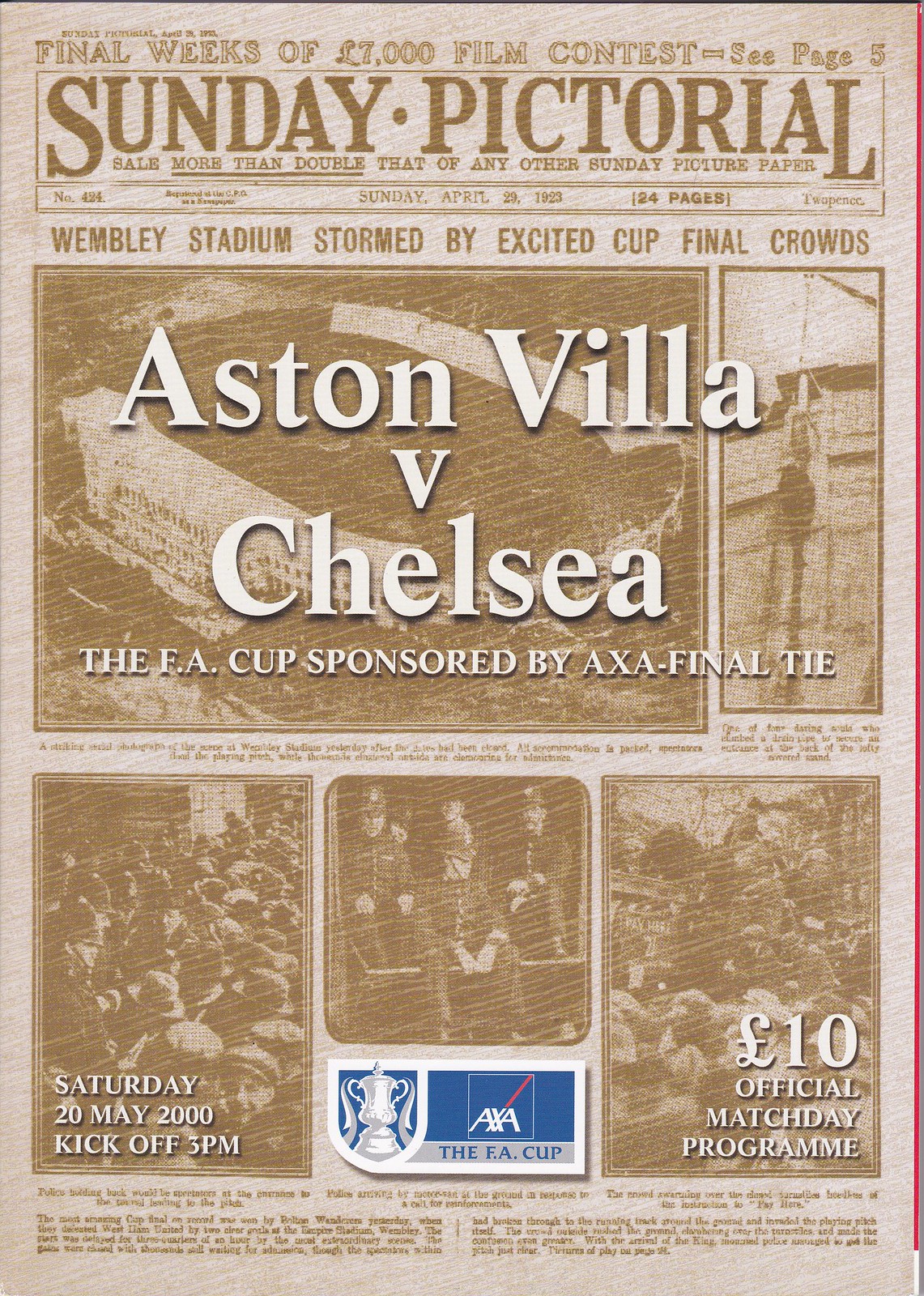The front page of the Sunday Pictorial dated Sunday, April 29, 1929, features a sepia-toned background with darker sepia text and images. At the top, it prominently announces "Final Weeks of 7,000-lb Film Contest, see page 5." Below this, the newspaper's title is displayed: "Sunday Pictorial - Sale More Than Double That of Any Other Sunday Picture Paper." The date and page count "24 pages" are noted alongside this. A significant headline reads, "Wembley Stadium Stormed by Excited Cup Final Crowds," referring to the FA Cup Final between Aston Villa and Chelsea. The event is scheduled for Saturday, May 20, 2000, with a kickoff time of 3 pm, sponsored by AXA, as indicated in white text over an image of the stadium. Below the stadium picture, three smaller images show crowds of people. The bottom left of the page mentions, "10-lb Official Match Day Program."